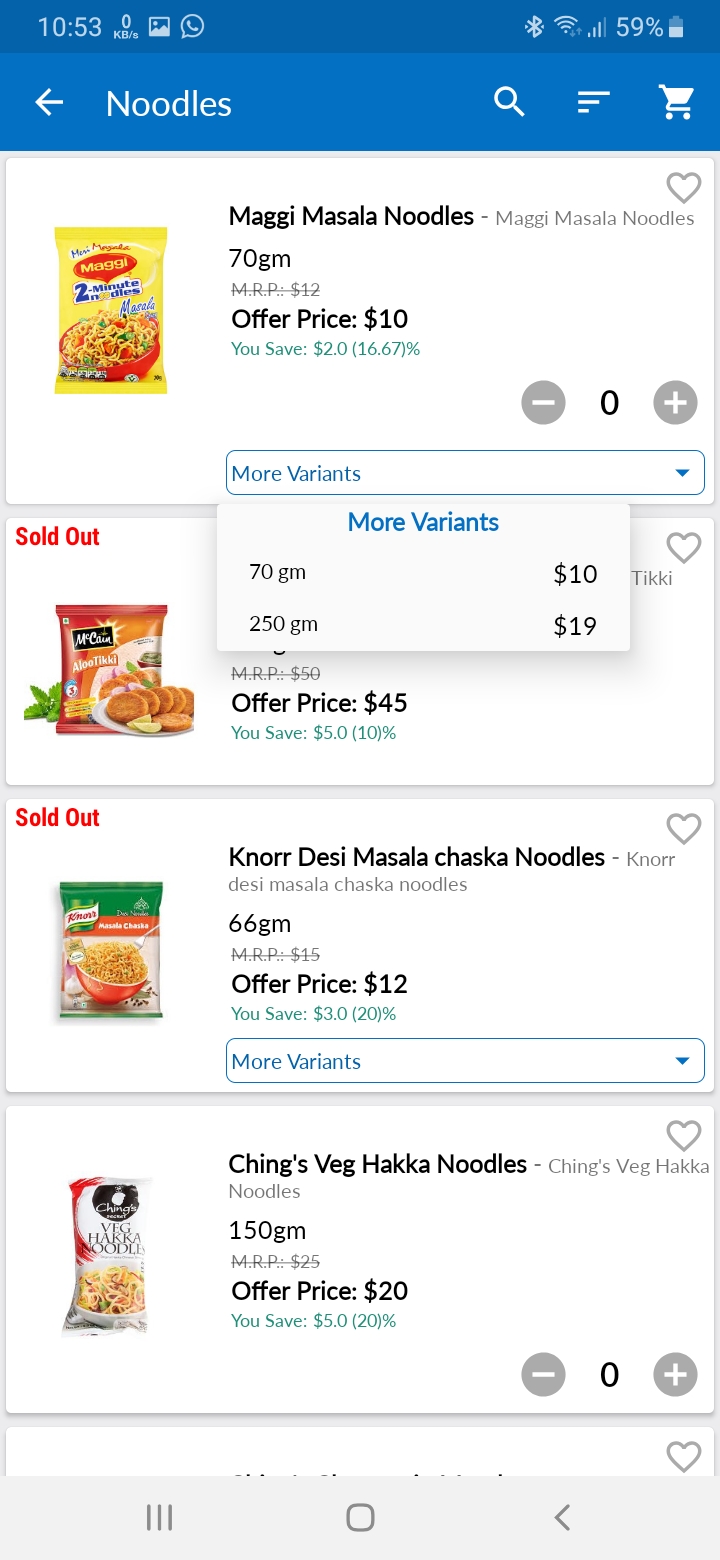**Detailed Descriptive Caption:**

The screenshot captures a smartphone screen displaying an online shopping app interface. The current time is 10:53, and the phone battery is at 59%. The Wi-Fi signal strength is shown with three bars, indicating a stable connection. The screen is focused on a search result page for noodles, featuring various noodle brands with their prices and quantities.

At the top of the list, "Maggie Masala Noodles" is highlighted. The 70-gram pack is available for $10, with an option to view more variants, including a 250-gram pack priced at $19. This section allows you to click on a heart icon to "like" the item and add it to a wish list.

The second item displayed is from an unknown brand, potentially "McCain," with an offer price of $45 marked as sold out. Below that, "Noor Desi Masala Kashka Noodles" by Noor is listed at $12 for a 66-gram pack, with additional size variants available.

Lastly, "Ching's Veggie Hakka Noodles" are available for $20 for a 150-gram pack, without additional size options. There is also a cart icon present, which is currently empty, and a magnifying glass for searching more items.